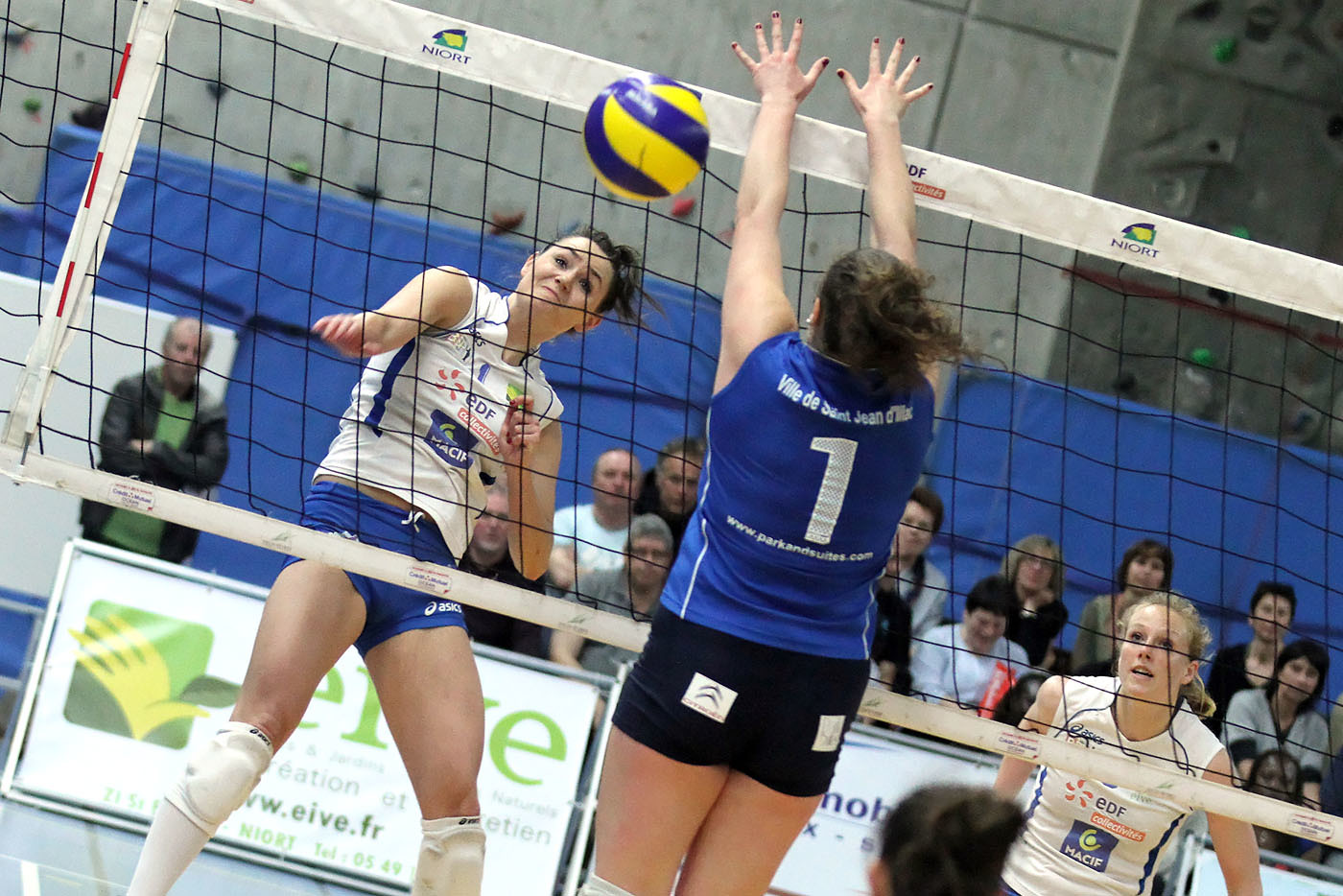In this detailed action photograph of a women’s volleyball game, the scene captures a tense moment as three players mid-air vie for control of the ball. In the foreground, a player in a blue and white jersey with the number one on the back, paired with black shorts adorned with white symbols, is positioned with both arms raised, her fingers outstretched, ready to hit the yellow and blue ball that hovers just below her hands. On the opposite side of the net are two players in matching white jerseys with extensive printing on the front, blue shorts, white knee pads, and white socks, appearing as if they have just sent the ball over the net. The photograph is slightly slanted from the upper left to the lower right, but the net remains prominently visible with some printing on its top white band.

In the background, spectators fill the bleachers, primarily older individuals intently watching the game, indicating the significance of the event—likely a high school or college tournament given the competitive atmosphere. Visible behind the bleachers are pads attached to a large concrete wall, providing both protection and a boundary for the play area. Separating the court from the spectators, railings are decorated with banners that add to the vibrant, energetic scene. A large piece of blue plastic tarp forms part of the backdrop, possibly used for tournament branding or additional containment around the court. The combined elements of athleticism, competition, and vibrant environment culminate into a vivid portrayal of the intensity and excitement inherent in a volleyball game.